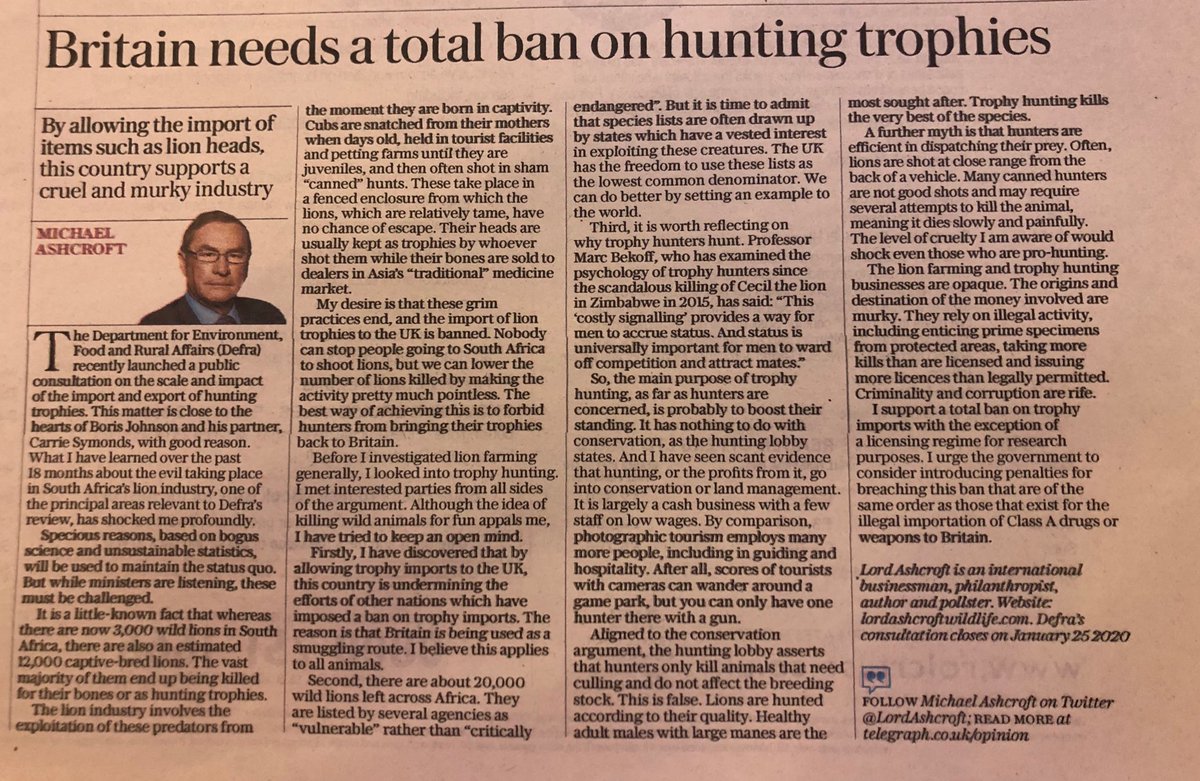A detailed newspaper clipping photograph reveals a passionate plea for a ban on hunting trophies. At the top, bold black text declares, "Britain needs a total ban on hunting trophies." Following this headline, an assertion critiques Britain for allowing the importation of items like lion heads, thereby supporting a cruel and murky industry. 

The article is accompanied by an image of a man wearing white glasses, identified as Michael Ashcroft by red text next to his face.

The black text continues, detailing that the Department of Environment, Food and Rural Affairs (DEFRA) recently launched a public consultation to assess the scale and impact of the import and export of hunting trophies. This issue holds significant importance for Boris Johnson and his partner, Carrie Simmons, due to good reason. Ashcroft shares his profound shock over the past 18 months spent learning about the horrific practices within South Africa's lion industry, a focal point of DEFRA's review. He condemns the suspicious motives founded on bogus science and unsustainable statistics used to uphold the current situation, asserting that these must be challenged by listening ministers.

The clipping further reveals a startling contrast: while South Africa harbors 3,000 wild lions, it also holds an estimated 12,000 captive-bred lions. Most of these captive lions face grim fates, often killed for their bones or as hunting trophies. The lion industry is described as exploiting these majestic predators, beginning when cubs are forcibly separated from their mothers just days after birth, confined in tourist facilities and petting farms until they mature, and then frequently subjected to being shot in staged hunts.

This emotionally charged article underlines the urgent necessity for a total ban on hunting trophies, advocating for the cessation of a barbaric industry.